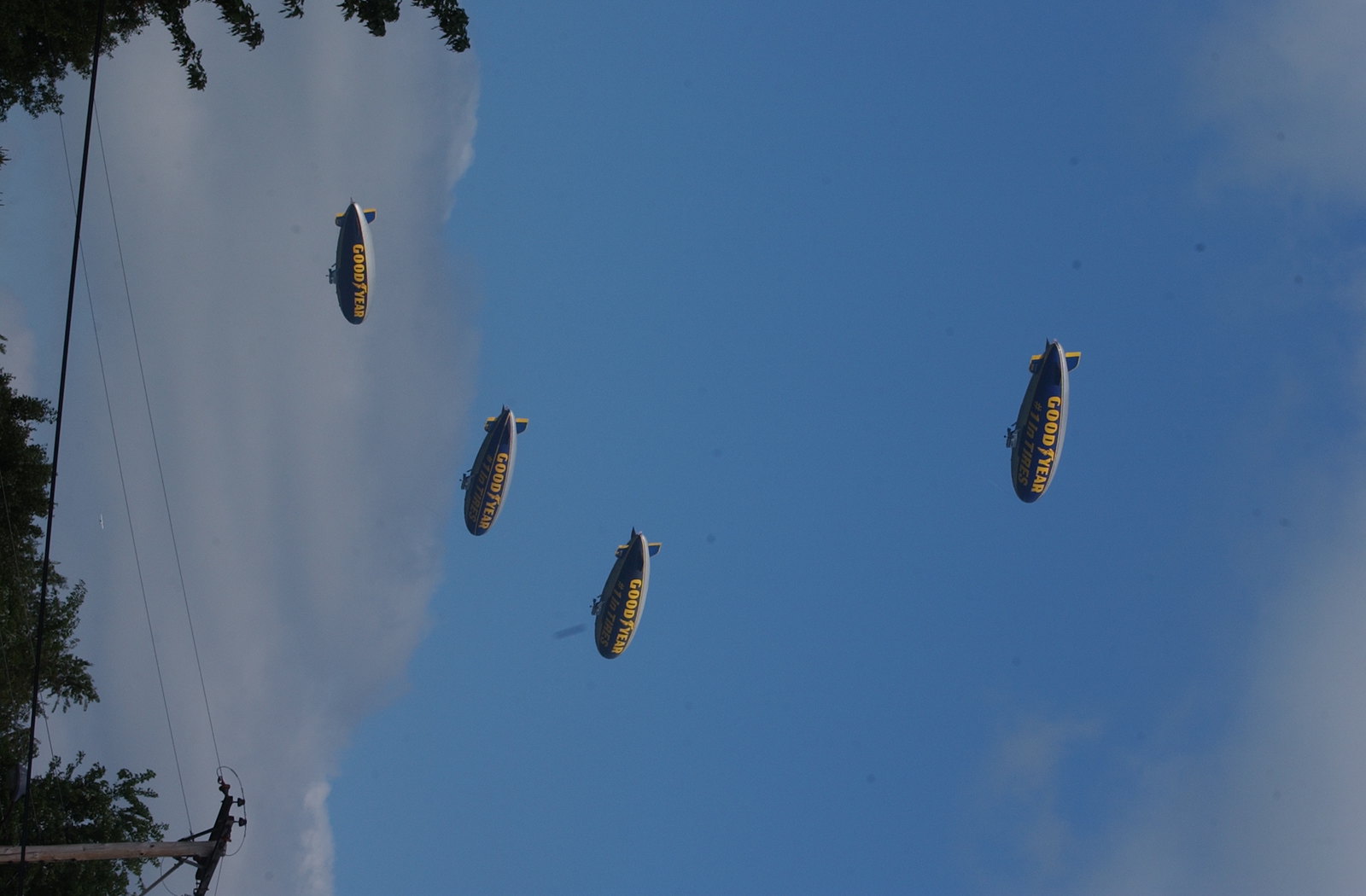This photograph, mistakenly oriented on its side, captures an aerial scene featuring four gray Goodyear blimps against a baby blue sky. The image requires a 90-degree rotation to the left for proper viewing. With a significant cloud formation gracefully dividing the sky, three blimps are positioned close together towards the lower left, and one is further up towards the top right, all bearing the distinctive yellow Goodyear logo. At what would be the bottom of the correctly oriented image, the tops of some trees and a telephone pole with visible wires are evident. The sky predominantly showcases a soft blue hue, with nuanced, funky cloud shapes adding character to the composition.